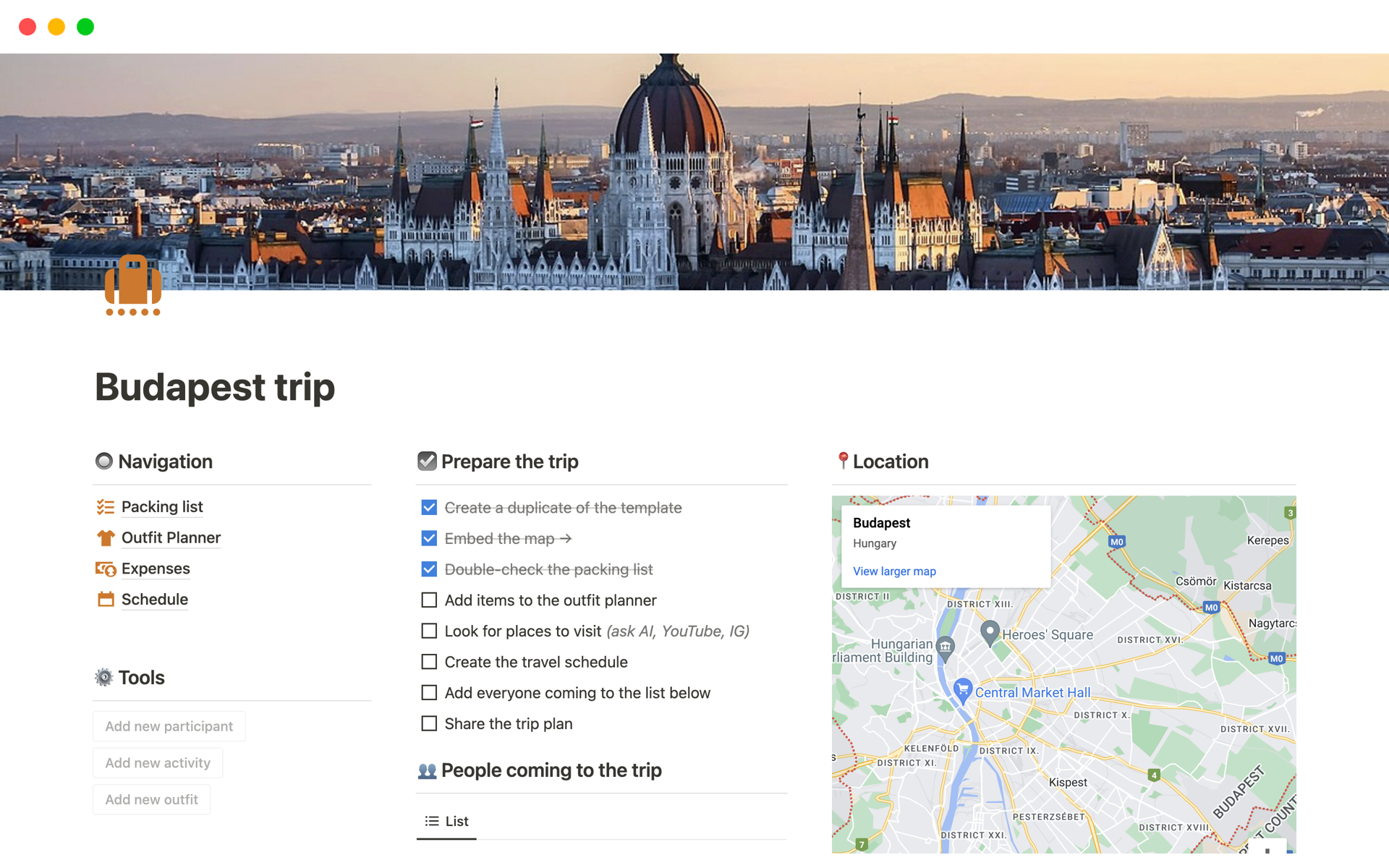The image is a detailed screenshot set against a white background, featuring a user interface likely related to trip planning, focused on a journey to Budapest, Hungary. In the upper right corner, three colored circles (red, yellow, and green) are visible. Below, there is a cityscape illustration, presumed to depict Budapest, which includes a large white building with a steep brown roof, possibly a historic church.

To the right, textual elements in black include the title "Budapest trip," followed by a list of sections: "Navigation," "Packing list," "Outfit planner," "Expenses," "Schedule," and "Tools." Below this, in gray text, are options such as "Add new participant," "Add new activity," and "Add new outfit."

Centrally placed in black text is the directive "Prepare the trip," followed by various tasks. Strikethrough gray text highlights completed actions such as "Create a duplicate template," "Embed the map," and "Double check the packing list." Remaining tasks in black text include "Add items," "Outfit planner," "Look for places to visit," "Create the travel schedule," "Add everyone coming to the list below," and "Share the plan."

Further down, in darker black text, is the section “People coming on the trip,” followed by a highlighted list of individuals. Accompanying this is a Google Map embedding, showcasing the location in Hungary, complete with road grades, highlighted yellow routes, and city names in black.

Overall, the image captures a thorough planning interface for an exciting trip to Budapest.